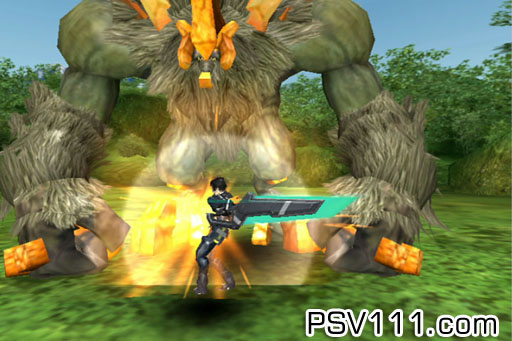In this action-packed image from a video game, a courageous character is depicted in the midst of an intense battle with a colossal monster. The character wields an enormous sword, with a distinctive black hilt and a vibrant green blade, which appears almost too large for her, yet she handles it with remarkable ease and determination. The towering monster, with its bulging, formidable muscles, stands approximately three to six times taller than the character, emphasizing the overwhelming challenge she faces. In the bottom right corner of the image, the text "psv111.com" is visible.